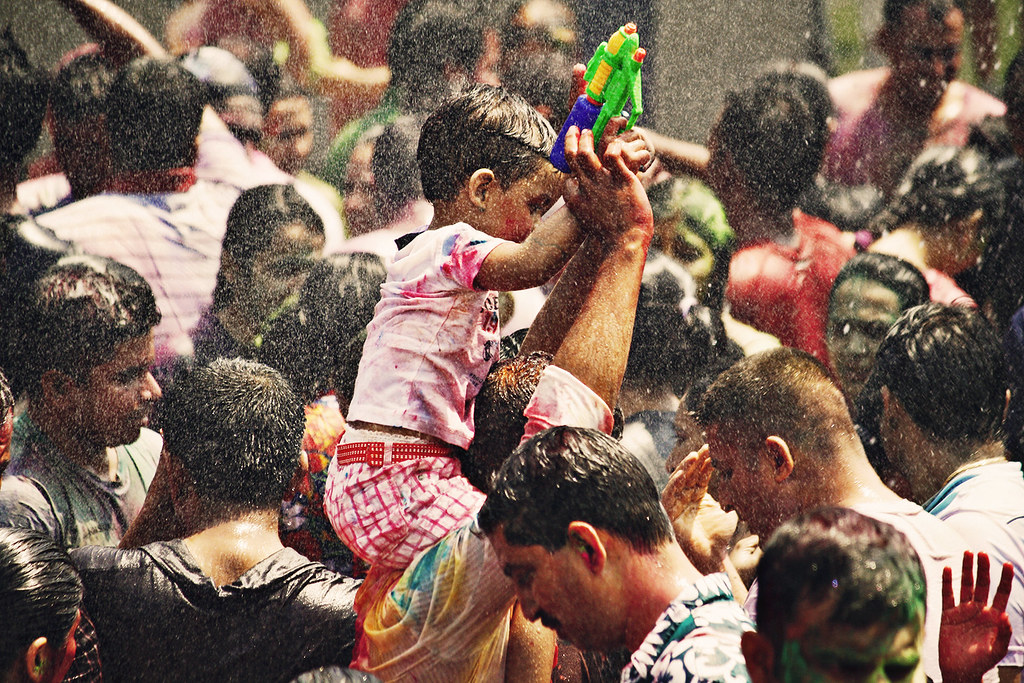The photograph is a rectangular color image, oriented vertically, capturing a vibrant and dynamic scene of a crowd of people, apparently of Indian descent. The majority of the individuals visible are sporting black hair and are clad in short sleeve shirts, creating a sense of casual uniformity.

Dominating the scene is a man wearing a colorful shirt with a small child perched on his shoulders. The child stands out prominently with a distinct outfit: a pink shirt splattered with a variety of colors, and red and white striped pants. He is also seen holding a vivid water gun, which features a blue water tank and green body with yellow accents.

There is a palpable sense of activity and movement among the crowd, with people appearing to be going in different directions. The foreground of the photograph is speckled with numerous water droplets, contributing to a lively atmosphere as if the scene is being showered upon, suggesting either celebratory water play or rainfall. The diverse reactions and the wet appearance of the crowd add layers of excitement and festivity to the image.